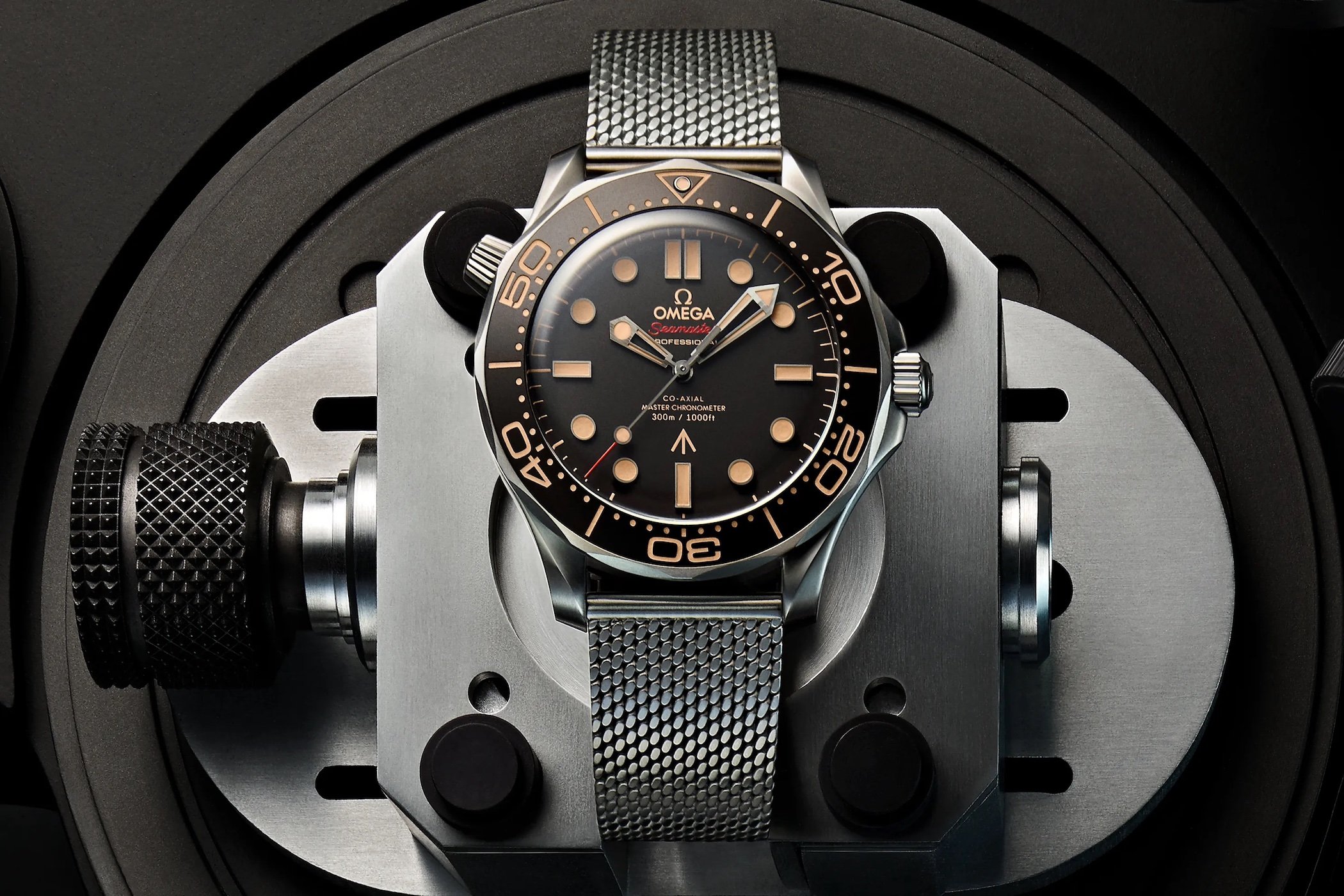This close-up photograph showcases a sophisticated Omega wristwatch, securely fitted into a watchmaking or jeweler's fixture, evidently designed for detailed work or adjustments. The watch itself is encased in a robust stainless steel housing, complemented by a sleek black dial and a functional steel mesh band, exuding an air of masculinity and durability.

Prominently displayed on the dial is the Omega brand name and the Greek symbol, both presented in a distinctive yellowish light brown color. The dial features indices represented by luminous dots and numbered segments in 10-second increments around the bezel, from 0 to 60, enhancing its precision and readability. The watch face is equipped with two substantial hands for the hour and minute, and a second hand with a subtle red tip, ensuring accurate timekeeping.

The watch is mounted on a square metallic base, part of a larger, intricate fixture. This apparatus, likely composed of steel, is connected to a circular base, intended for stability and maneuverability, possibly allowing the watch to be rotated or adjusted precisely. The fixture includes a black dial, possibly for adjusting the position, with lines indented on the circular platform, hinting at a track mechanism for seamless rotation, further aiding the craftsman's work.

Overall, this image merges elegance and functionality, capturing not just the refined aesthetics of the Omega wristwatch but also the meticulous environment of horological craftsmanship.